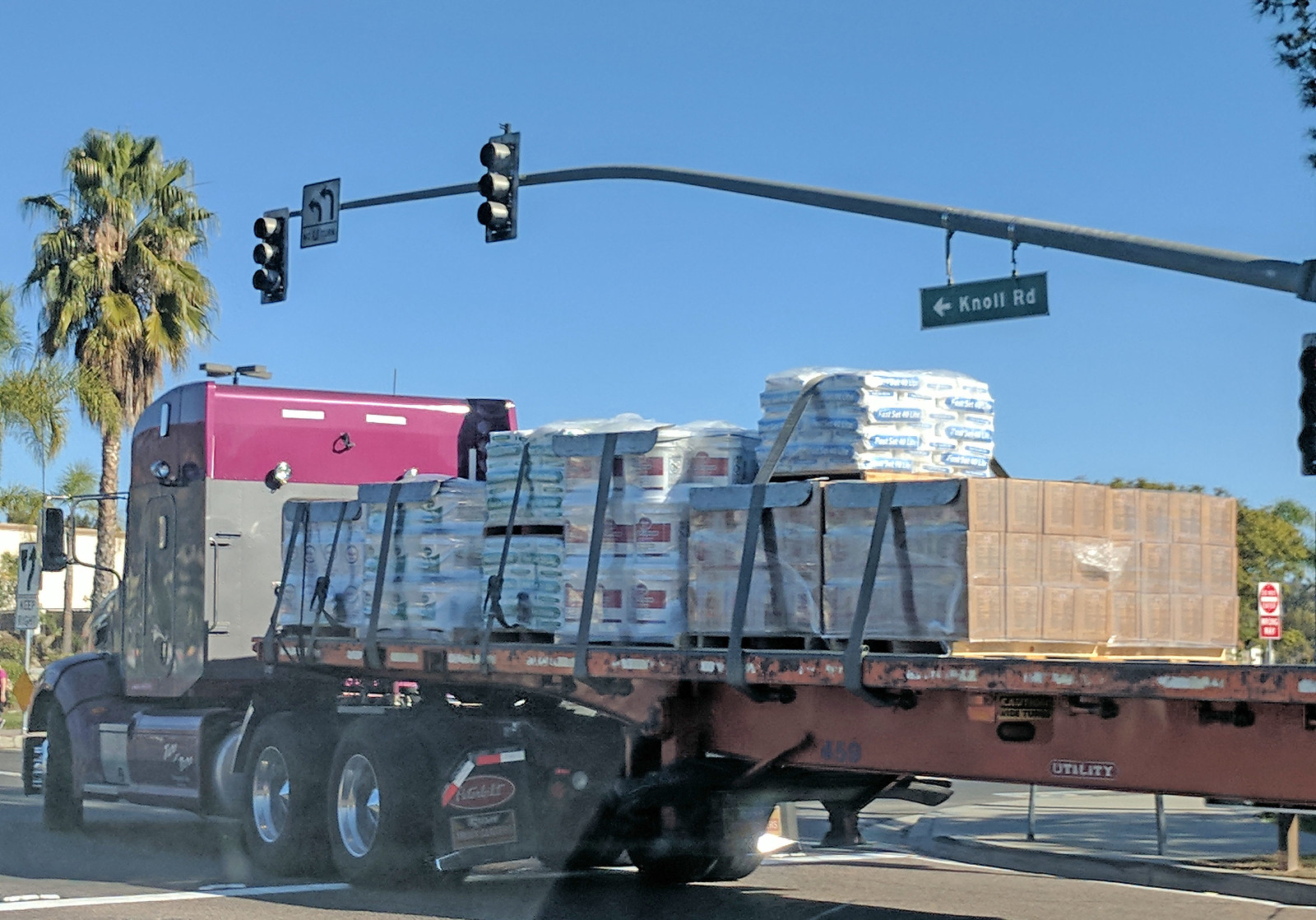An 18-wheeler truck with a flatbed trailer is navigating a right turn at the intersection of Knoll Road on a sunny day under a clear blue sky. The cab of the truck features a red top and a beige bottom. The flatbed trailer, open-faced without walls, is tightly packed with a variety of heavy items. These include large white packages, two big brown containers, likely bags of cement, plastic-wrapped pallets with large buckets, and other stacked rectangular boxes that form a grid near the back of the trailer. The cargo is secured with wide nylon straps. The truck is halfway through the intersection, with its wheels turned right. The intersection is wide, marked by an extensive traffic light post that supports multiple sets of signal lights and double turn lane signs. The backdrop features tall palm trees, enhancing the distinctly sunny landscape.